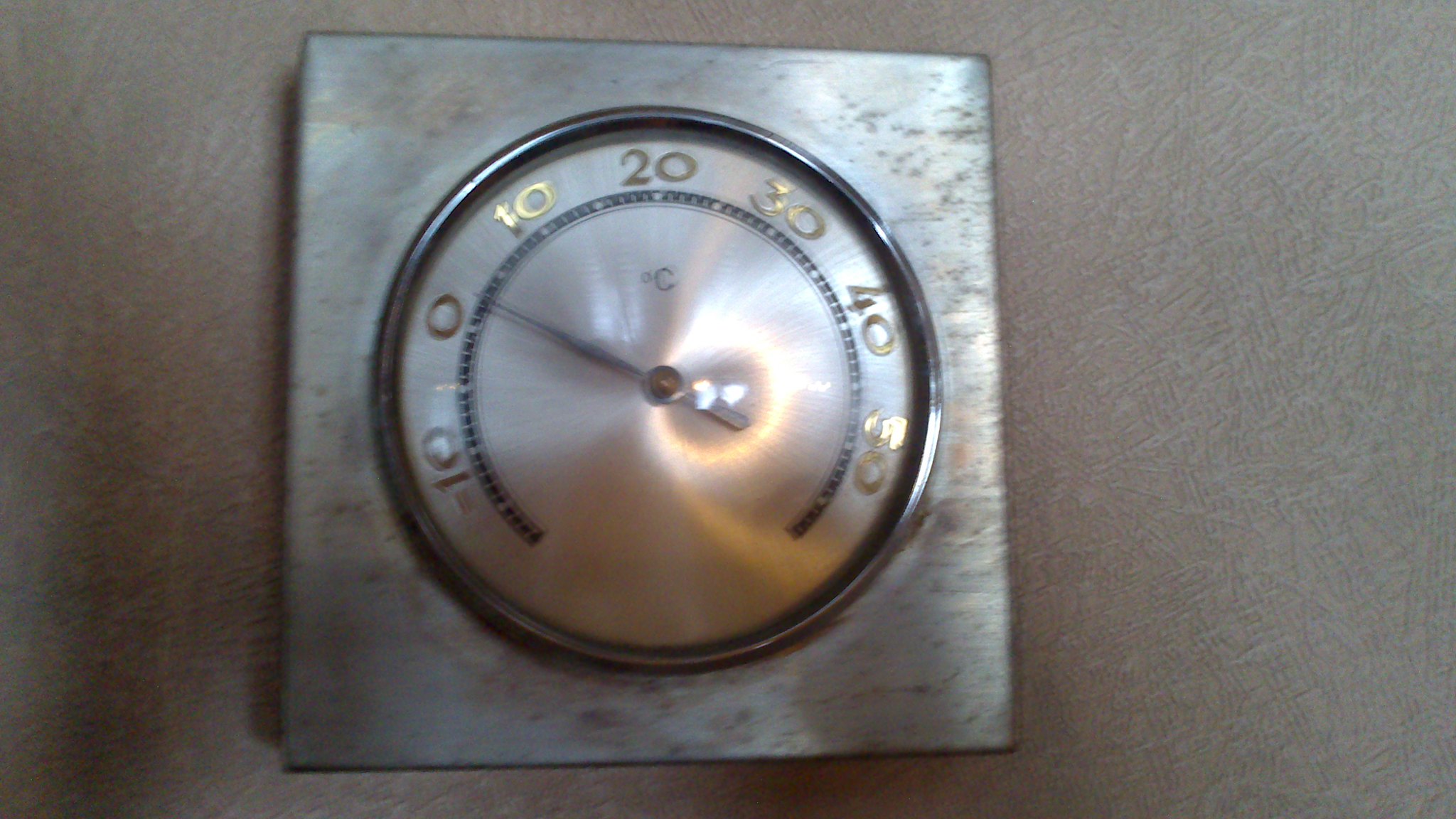The image depicts a classic round thermostat mounted on a slightly worn and oxidized white wall, which appears darker due to the lighting. The thermostat features a silver plate and a circular bezel, creating a sophisticated frame around the temperature dial. The temperature display ranges from -5 to 55 degrees Celsius, and currently, the needle, which is also silver, points to around 2 or 3 degrees Celsius, indicating the current room temperature. The numbers on the dial are in a darker silver, providing clear contrast and legibility against the lighter silver background. The thermostat may simply show the temperature rather than allow for adjustments, adding a vintage charm to its functional design.